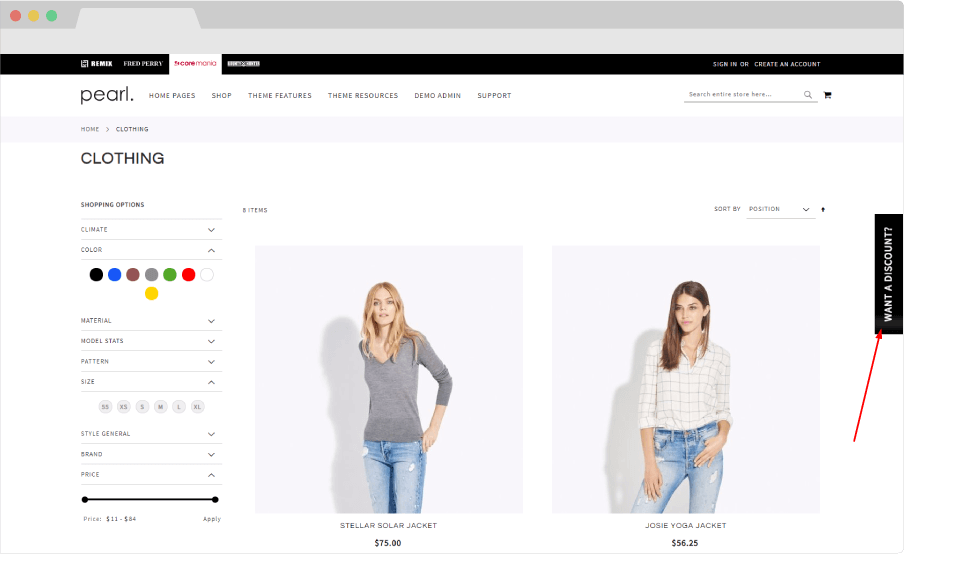Here is a detailed and cleaned-up caption for the image:

---

This screenshot showcases an e-commerce website focused on selling clothing. At the top of the page, a gray border features three small circles in the upper left-hand corner, colored red, yellow, and green in sequence. Below this is a blank gray area, representing where the address bar would typically be displayed. 

The next section down features a black border with mostly unreadable text; however, on the far right, there is an option to "Sign In or Create an Account." Directly beneath this border is a navigation bar labeled "Perl, Home Pages, Shop, Theme Features, Theme Resources, Demo Admin, and Support," with a search bar and shopping cart icon situated to the right.

The main part of the page is dedicated to clothing, specifically the "Clothing" category. Shopping options include several selectable filters such as Climate, Color, Material, Model Stats, Pattern, Size, Style General, Brand, and Price.

On the right-hand side of the page, a prominent red arrow points to a black box with white text reading "Want a Discount?" Below this promotional message are images of two young women modeling clothing. 

The first woman, with blonde hair, is wearing blue jeans and a gray shirt, labeled as "Stellar Solar Jacket" priced at $75. The second woman, sporting brown hair, is dressed in a plaid shirt and blue jeans, identified as "Josie Yoga Jacket," available for $56.25.